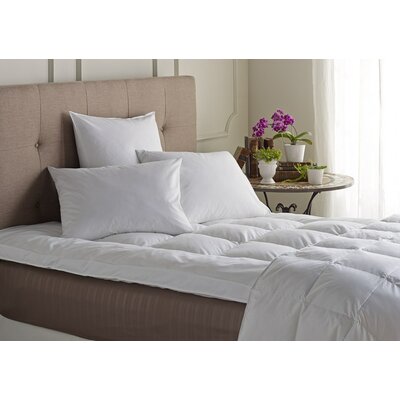This image captures a meticulously maintained bedroom with an air of upper-middle-class elegance, possibly reminiscent of a hotel room. The centerpiece is a bed adorned with a beige fabric headboard and base, complemented by a white quilted duvet cover. Three fluffy white pillows are neatly arranged against the headboard, adding to the sense of comfort and luxury. The wall behind the bed features a distinctive wainscoting design in a creamy white hue. To the right of the bed, natural sunlight filters through sheer white curtains, enhancing the room's bright and inviting ambiance. A small circular table stands next to the bed on the right side, showcasing three potted plants, two of which are adorned with delicate pink flowers.